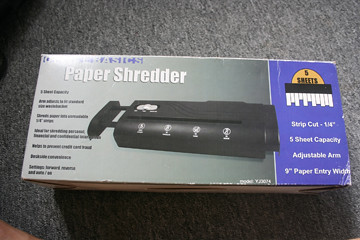The image portrays an amateur, colorized photograph of a paper shredder's packaging, situated on a slightly bent, horizontal box, displayed on a tight, gray office carpet, in a dimly lit room. The cardboard box prominently features marketing text and images that detail the shredder’s specifications, including a black shredder depicted with various functional buttons in white. On the right side of the box, highlighted by a purple strip, are specific details: "5 sheets, strip cut, 1/4 inch, 5 sheet capacity, adjustable arm, and nine-inch paper entry width." Additionally, there is a section with unreadable text and icons that presumably describe further functions and features, but these are too small and indistinct to decipher. The brand "Basics" is also visible on the box.